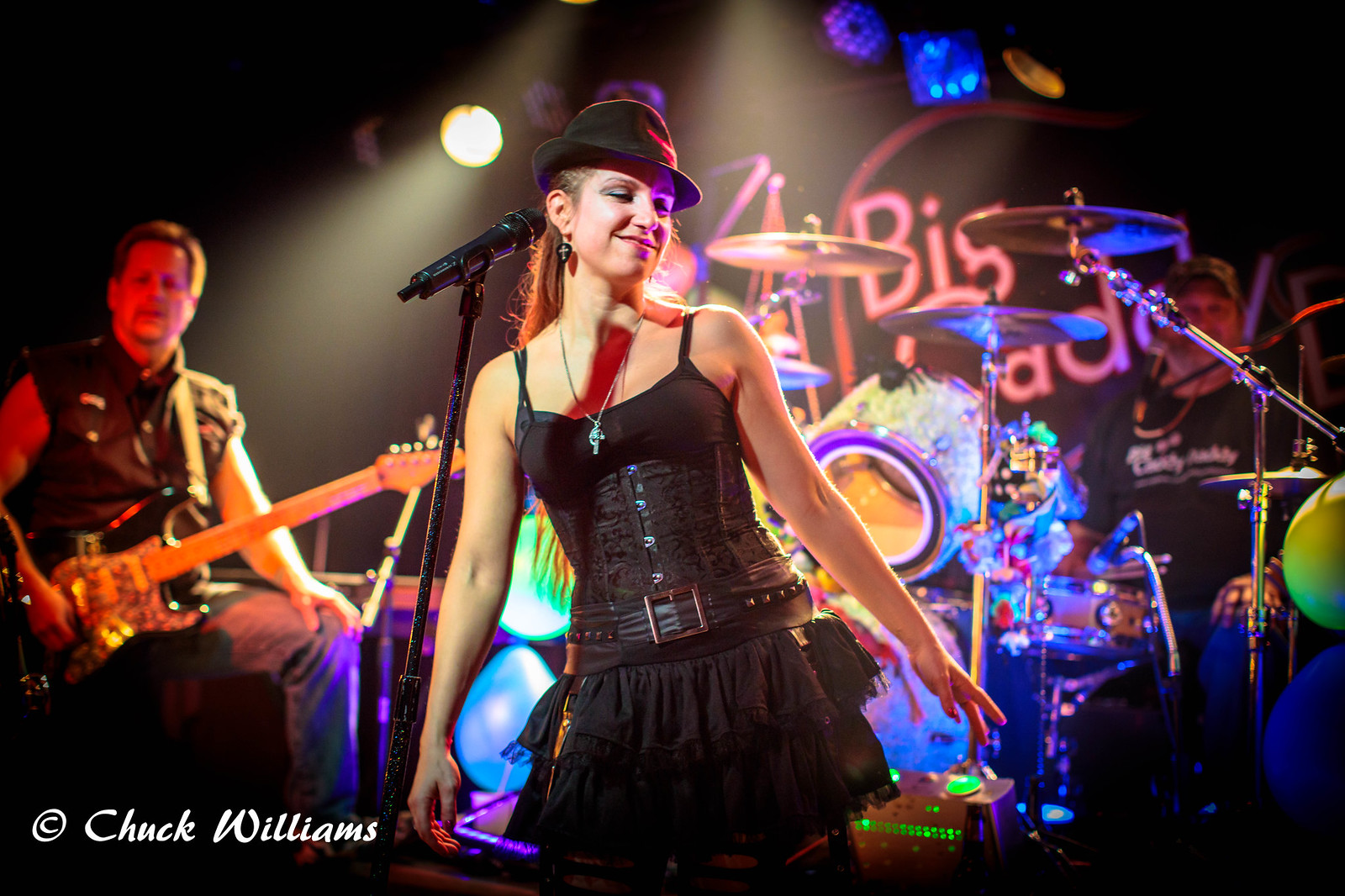This horizontal rectangular image captures an engaging live band performance. Dominating the foreground is the lead singer, a woman standing confidently in front of a stand-up microphone. She is dressed in a black spaghetti-strap dress cinched at the waist with a belt, and her hair flows freely down her back. She dons a stylish hat and has a smile on her face, exuding charisma as her arms extend down by her sides.

To her right, partially in the background, is a guitarist with brown hair and wearing a brown shirt. His guitar is strapped over his shoulder, but he's momentarily resting his hand on his knee, suggesting a brief pause in playing. On the far right, in the distant background, a barely visible figure in a black t-shirt and green hat can be seen.

Behind the singer, the drummer and his vividly colored drum set, featuring blue, purple, and pink cymbals, add a dynamic visual contrast against the darker backdrop. Various microphones are scattered around, and above them, a few neon signs illuminate the space. A ceiling fan with a light fixture is also visible, and to the left, the subtle appearance of the moon adds an atmospheric touch. The lower left corner of the image credits "Chuck Williams" as the photographer, completing the scene.